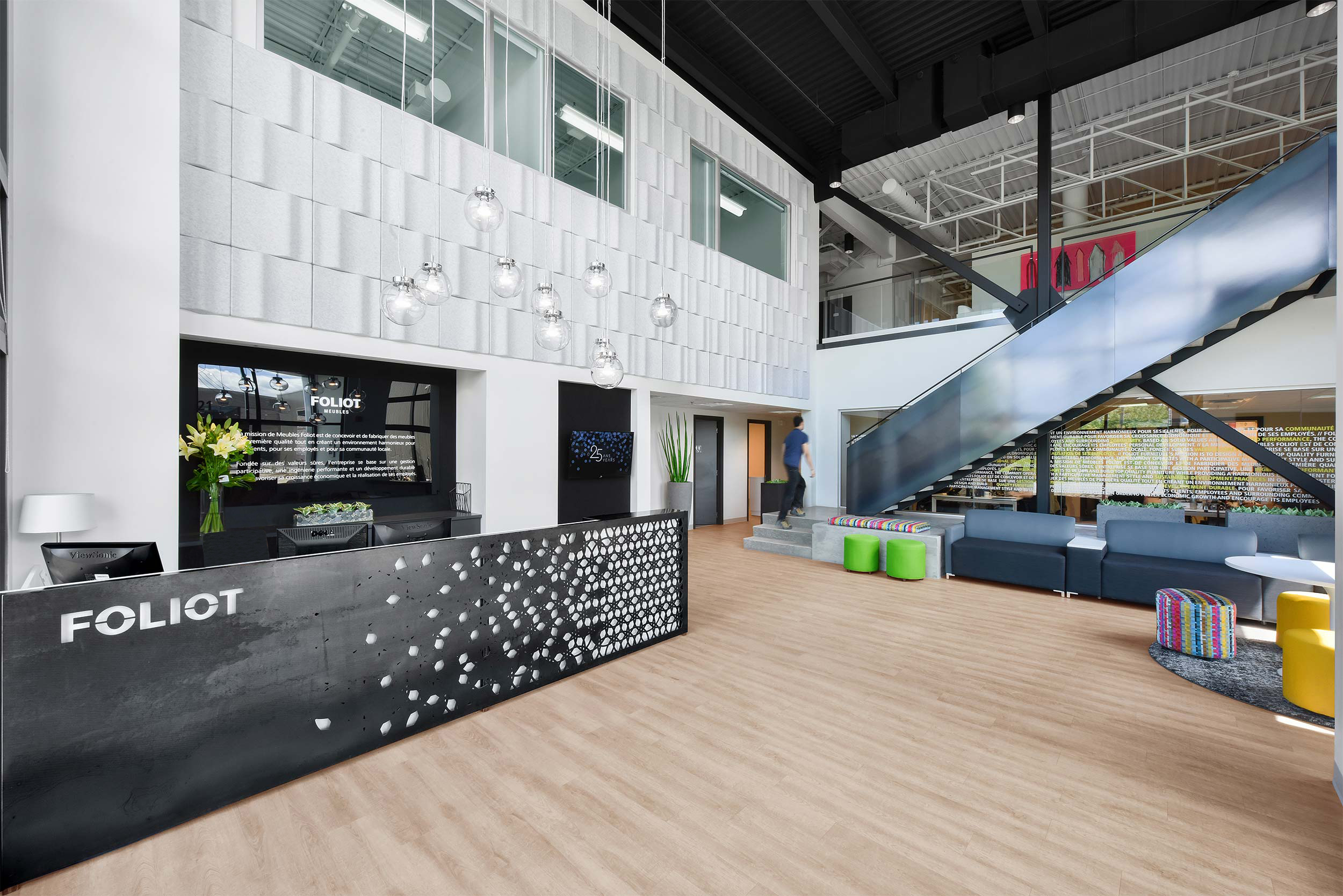The image depicts the interior of a modern, upscale office or studio building branded as "FOLIOT," with its name prominently displayed in bright white block letters against a black backdrop that has a design resembling small white dots or petals. The setting appears to be both a reception area and an inviting lounge space. Upon entering, on the left side, there's a sleek reception desk with a black countertop, behind which are visible computers and a large white planter housing a green plant. The entry area is defined by light brown flooring and is accented by various white and chrome elements.

In the background, a metallic staircase ascends to the next level, and underneath it, there's a cozy seating area featuring lime green chairs, sofas with matching footstools, and a small table with additional seating, suggesting a casual spot for discussions or breaks. Directly in front of the reception, a variety of seating options are available, including single chairs and couches, all designed for comfort. The entire space is well-lit, with bulbs hanging down from the high ceiling, casting a warm, welcoming glow throughout.